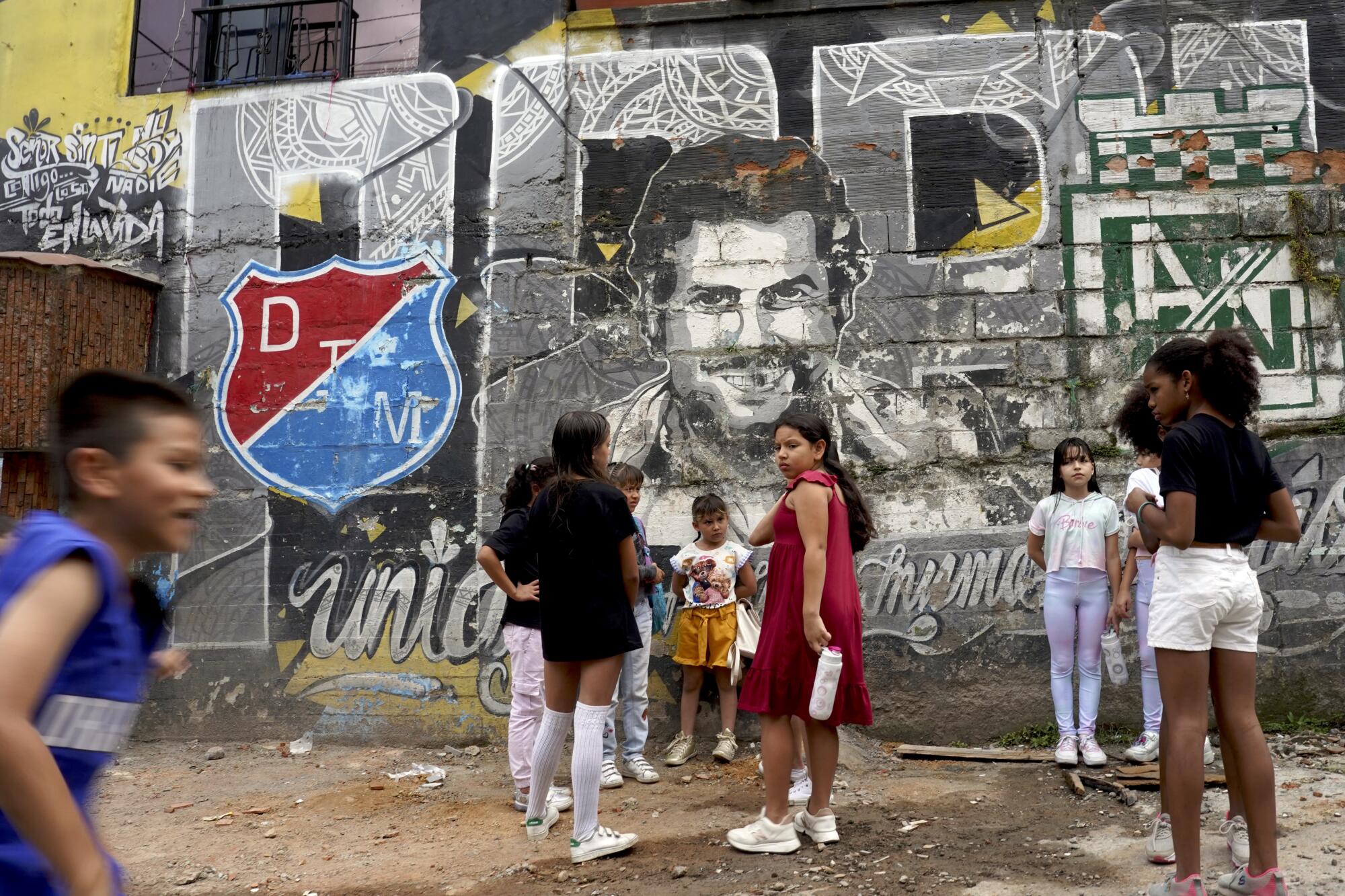The photo captures a mural honoring the infamous drug lord, Pablo Escobar, on the side of a building in a slum area. The image, which is square and taken outdoors during the day, features a large, colorful portrait of Escobar smiling at a group of children. The mural is decorated with graffiti and partially legible letters, including "DTM" on a blue and red shield. The ground is a dirt patch scattered with rocks and trash. In the lower left corner, a young boy in a blue tank top or jersey is visible in motion, and near him, a young black girl wearing white shorts and a blue top. Surrounding them are other children, mostly Hispanic, with dark hair, some wearing shorts, dresses, or light-colored skinny jeans. The scene is a chaotic blend of vibrant colors including black, maroon, various shades of blue, light purple, white, green, yellow, brown, and light brown. Some children are looking directly at the camera, while others are not, highlighting the mixed emotions and everyday reality in the backdrop of this unsettling homage.